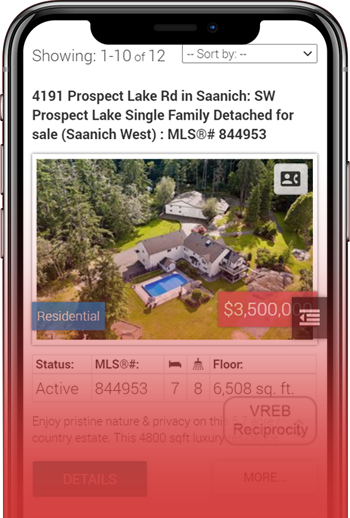The image features the top half of a shiny black phone with a web page displayed on its screen. The phone has rounded edges and silver metallic power and volume buttons on the left side, with an additional button on the right side. The top margin of the screen has a half-rectangle with rounded edges, containing a central speaker and a bluish camera lens to the right. The web page on the screen is a realty listing with a white background. At the top, thin light gray text reads "Showing 1 through 10 of 12" followed by a rectangular drop-down box with gray text reading "Sort by". Below, in bold black text, is the listing title "4191 Prospect Lake Road in Saanich SW, Prospect Lake Single-Family Detached for Sale" and in brackets "Saanich West MLS R# 844-953". Underneath, a color aerial photo shows a home with a pool, large expanses of green grass, and is surrounded by bright green pine trees. A blue label in the bottom left corner reads "Residential", and a red label in the bottom right corner displays "3,500,000".